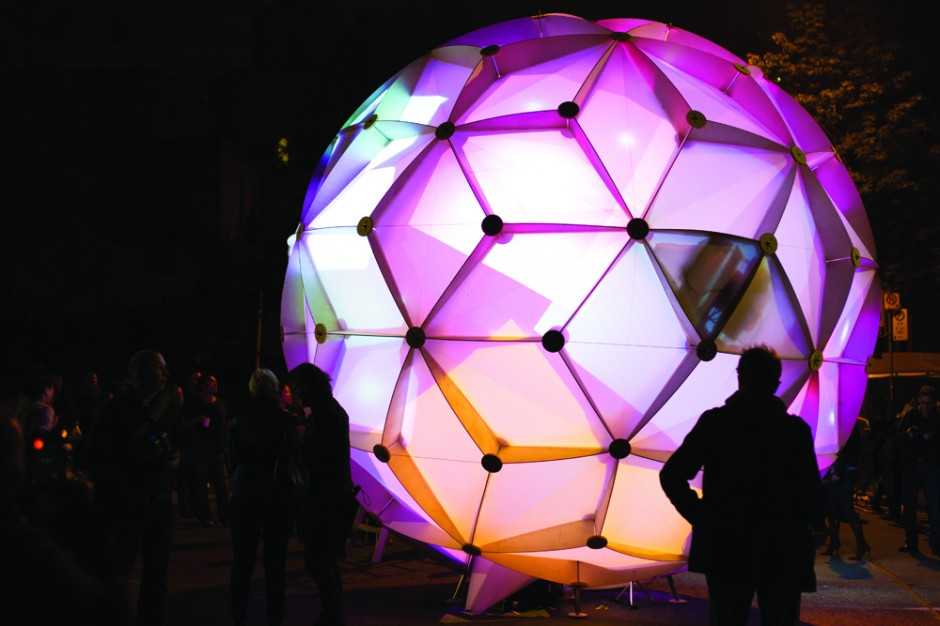The photograph captures a captivating outdoor scene at night featuring a large, illuminated orb towering over a small group of silhouetted onlookers. The orb, resembling a monumental New Year's Eve ball, radiates a kaleidoscope of vibrant colors including purples, oranges, greens, blues, and pinks. It consists of geometric panels, primarily hexagonal and diamond-shaped, with distinctive black joint patterns resembling flowers, giving the ball a textured, three-dimensional appearance. Dominating the foreground is the silhouette of a man with short, spiky hair, possibly wearing a coat, with his arm bent as if placing his hand in his pocket. To the right, the soft lighting hints at the presence of a tree, while faint silhouettes of clustered individuals are visible on the left, set against the inky darkness of the background. This mesmerizing display of colors and shapes against the night sky draws attention to the art piece, standing approximately 15-20 feet tall and serving as an intriguing focal point for the gathering.